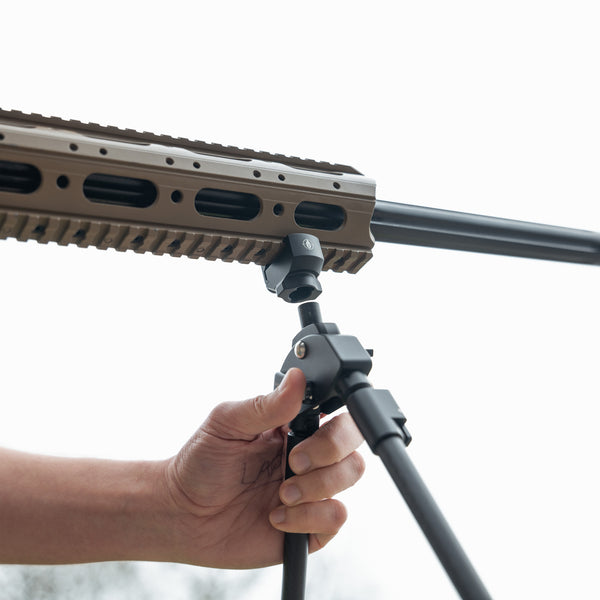The photo depicts a close-up scene in which a Caucasian male is attaching a black tripod to a rifle. The man's left hand is holding the tripod, which features a silver screw mechanism for attachment. Only part of the rifle, specifically half of the barrel, is visible, and it has a brown casing that's indicative of a modern firearm. The image is set against a completely white background, possibly hinting that the scene was shot with professional lighting to highlight the subject—giving the photo a catalog or advertisement feel. There is a blurred area suggesting the presence of trees, indicating the scene could be outdoors, though the background remains predominantly white. The image is detailed, with clear emphasis on the hardware and connection between the tripod and the rifle.